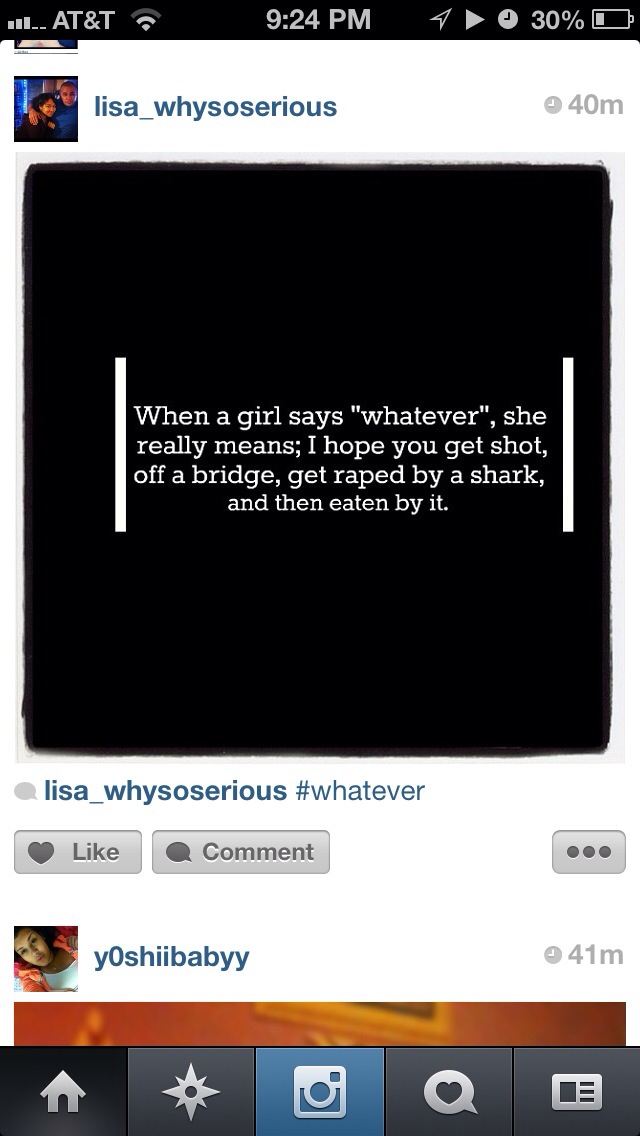The image depicts a mobile phone screen showing a social media app interface. At the top, the status bar is visible, indicating AT&T service, Wi-Fi connectivity, the time (9:24 p.m.), and a 30% battery life. The screen displays a post from the user "Lisa_why_so_serious," created 40 minutes prior. The post features a stark black background with white text that reads, "When a girl says whatever she really means, I hope you get shot off a bridge, get raped by a shark and then eaten by it." The post includes two white lines on either side of the text. Below the post, there are options to like, comment, and access further actions through a three-dot menu. The bottom section of the screen showcases five icons, indicating navigation options for different modules of the app. Additionally, there is an adjacent post from another user, with their details partially visible.